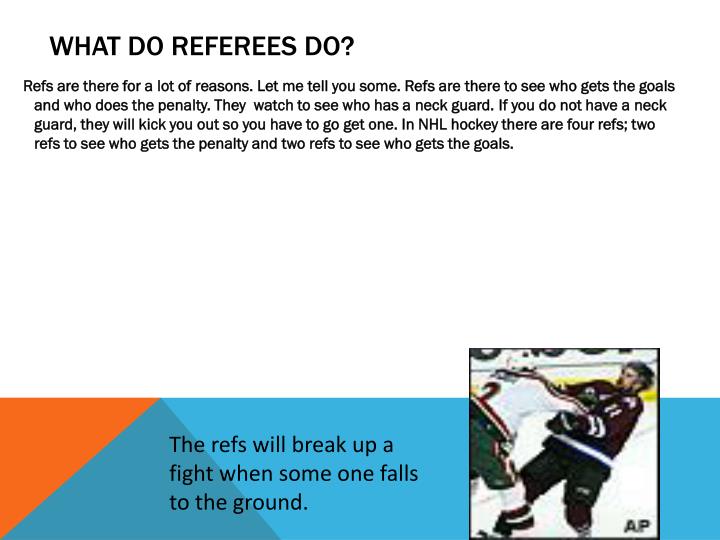The image displays a PowerPoint presentation slide primarily focused on describing the roles of referees in hockey. The slide's headline, "What do referees do," is followed by detailed black text explaining various duties: Referees are responsible for determining who scores goals and who incurs penalties. They also ensure that players wear neck guards, ejecting those who don't comply to enforce safety. Particularly in the NHL, there are four referees: two focused on penalizing infractions and two on awarding goals. At the bottom of the slide, within a blue rectangular bar with an orange corner, black text states that referees will stop a fight when a player falls to the ground. This text is accompanied by an image of two hockey players engaged in a fight on the ice, positioned towards the bottom right of the slide. The slide is set against a white background with various colors including black, blue, orange, maroon, and green.